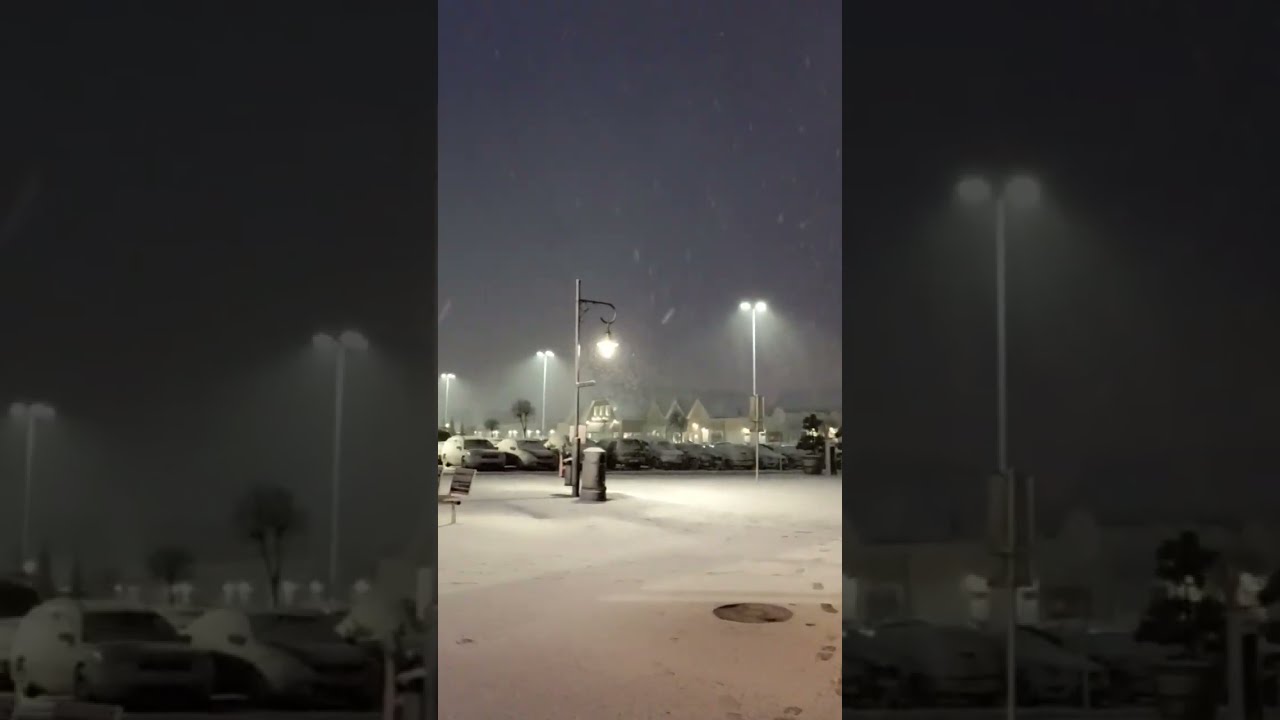This photograph captures a snowy nighttime scene in what appears to be a city parking lot or wide street, possibly part of a recreational area or shopping center. The ground is blanketed with fresh snow, accentuating a dark gray pavement with a visible sewer cap on the right. Light posts, illuminated and casting a gentle glow, line the area and add a subtle white hue to the otherwise dark, gray sky. There are several snow-covered cars arranged toward the center of the image, with a bench positioned to the left and a metal trash can near one of the light posts. In the backdrop, a row of houses or buildings is partially visible, giving context to the neighborhood setting. Footprints in the snow and scattered trees add depth and a sense of scale to the serene, wintry scene.